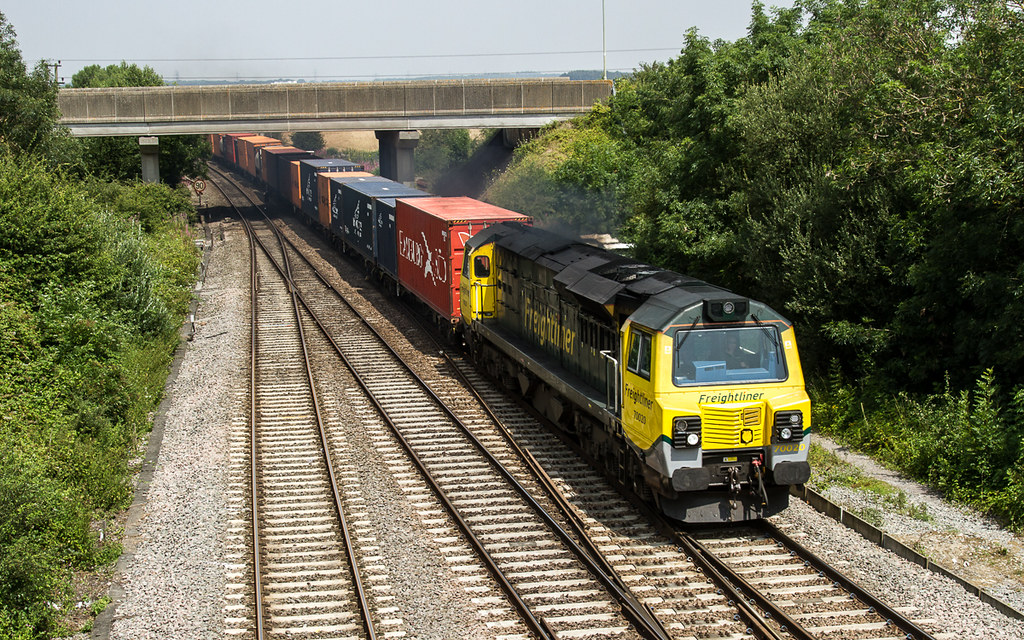The photograph captures a vivid scene of a freight train traveling along a multi-track railway. The front engine, prominently positioned at the bottom right, is a yellow and black locomotive marked with "Freight Liner." Wisps of smoke drift from the engine, adding a dynamic touch. The train stretches diagonally across the image from the bottom right to the top left, with its assorted cargo cars trailing behind in an array of colors—reds, blues, and oranges. The tracks multiply as they recede, expanding from two to four sets. Flanking the tracks, lush greenery with dense trees and bushes frames the scene on both sides. A cement bridge with built-up fence sides arches over the tracks toward the image’s right-center, accompanied by power lines and a hazy skyline that casts a bluish-gray light over the distant cityscape. The overall composition is rich with detail, capturing the movement and industrial strength of the passing freight train amidst its natural and urban surroundings.